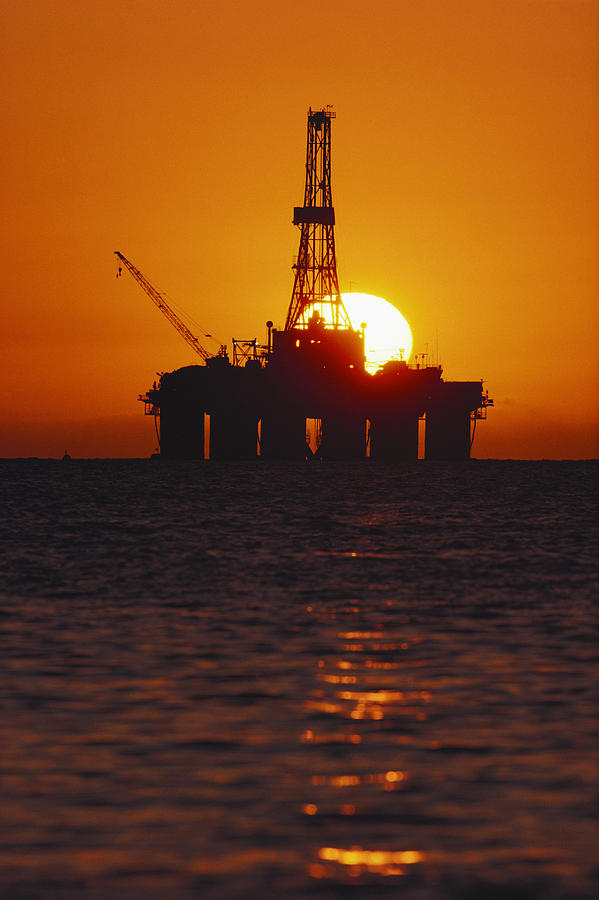This photograph captures an offshore oil drilling platform silhouetted against the setting sun. The platform, reminiscent of the Eiffel Tower with its skeletal steel structure, stands supported by six concrete pylons embedded in the dark ocean waters. The sun, low in the sky, casts an orange glow across the entire scene, transforming the white caps of the waves into glistening gold. To the left, a crane with a hook at its end extends from the platform, adding to the industrial silhouette. The sunlight reflects off the water, enhancing the dramatic effect of the sunset behind this towering oil rig.